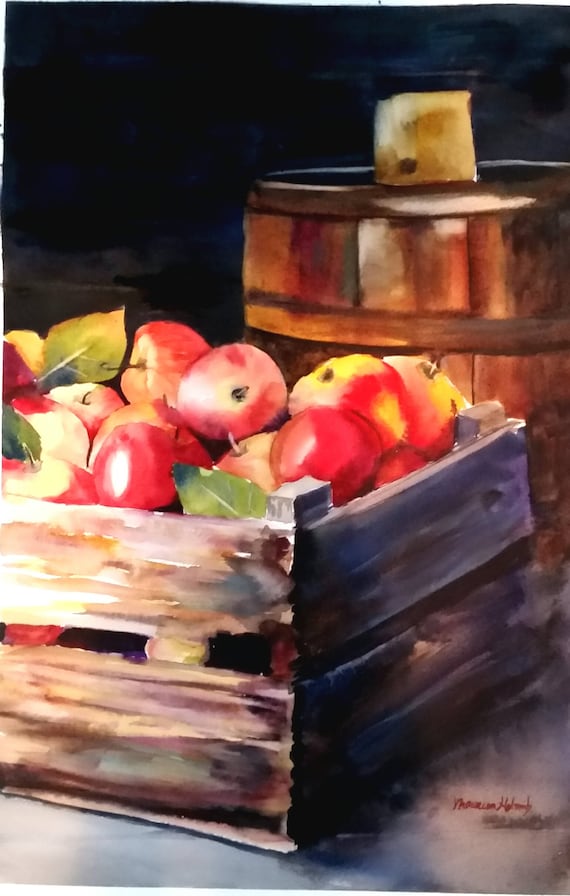This is a detailed watercolor painting featuring a square wooden crate brimming with apples in various shades of red, with some displaying golden patches. Scattered among the apples are a few leaves, adding a touch of nature to the scene. The crate appears to be somewhat weathered, reflecting a rustic charm. Positioned behind the crate is a brown wooden barrel with an indistinguishable object resting on top, possibly a piece of wood or cheese. Set against a very dark background, the crate and barrel stand out prominently, casting striking contrasts. The foreground features the crate perched on a grayish circle. In the bottom right corner, the painting is signed by the artist, though the signature is illegible.